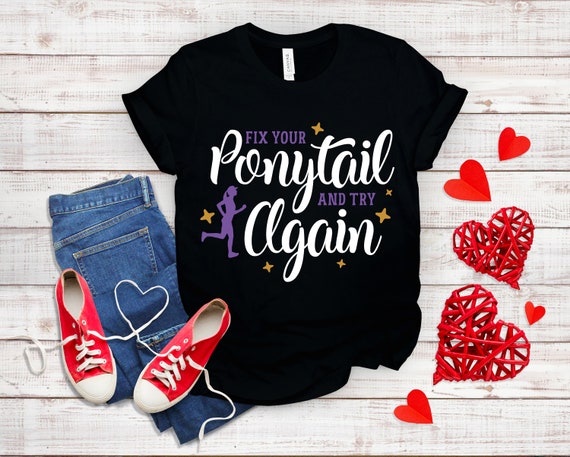The image is a staged, full-color advertisement for clothing, featuring a meticulously arranged setup on a distressed white wooden surface with visible horizontal lines separating the boards. The scene centers around a black t-shirt with the motivational phrase "Fix your ponytail and try again." The text includes a mix of purple and white colors: "Fix your" and "And Try" are in purple, while "Ponytail" and "Again" are in white cursive. Surrounding the words "And Try" and "Again," there are several yellow stars, and to the left of "Again" is a purple silhouette of a woman running. 

To the left of the t-shirt, a pair of blue jeans is partially folded with a pair of red Converse tennis shoes placed on them. The laces of the shoes are arranged to form a heart shape. On the right side of the t-shirt, there are several hearts made of what appears to be wood or paper mache, varying in size. The setup hints at a message of resilience and striving, targeting a female audience, with the distressed white wooden background adding a rustic charm.